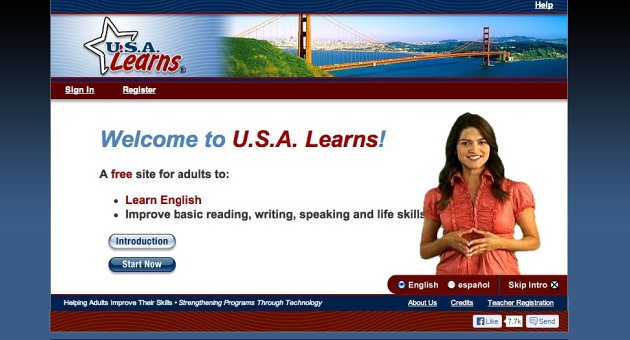The image depicts a dated, rectangular web page for "USA Learns," a free site designed to help adults improve their English reading, writing, speaking, and life skills. The top half features a banner with a black-to-blue gradient background, showcasing the "USA Learns" logo on the left and a help button on the right. Adjacent to the help button is an image resembling the Golden Gate Bridge, depicted in a golden hue over a large body of water with greenery on both ends. Below the banner, there is a maroon-colored navigation bar offering links to "Sign In" and "Register."

The main section of the page is white and includes a prominent welcome message: "Welcome to USA Learns, a free site for adults to learn English, improve basic reading, writing, speaking, and life skills." Accompanying this text on the right side is a photograph of a smiling woman with long dark hair, wearing a peach or coral-colored blouse. Just beneath this description are two buttons labeled "Introduction" and "Start Now."

The lower portion of the page includes options to view the site in either English or Español, and a "Skip Intro" button. Further down, there is a blue section with links to "About Us," "Credits," and "Teacher Registration." At the very bottom is a maroon section containing buttons for "Like" and "Send," along with text indicating "Helping adults improve their skills through technology." The main colors of the website are red, white, and blue, evoking a sense of patriotism fitting for the "USA Learns" theme.